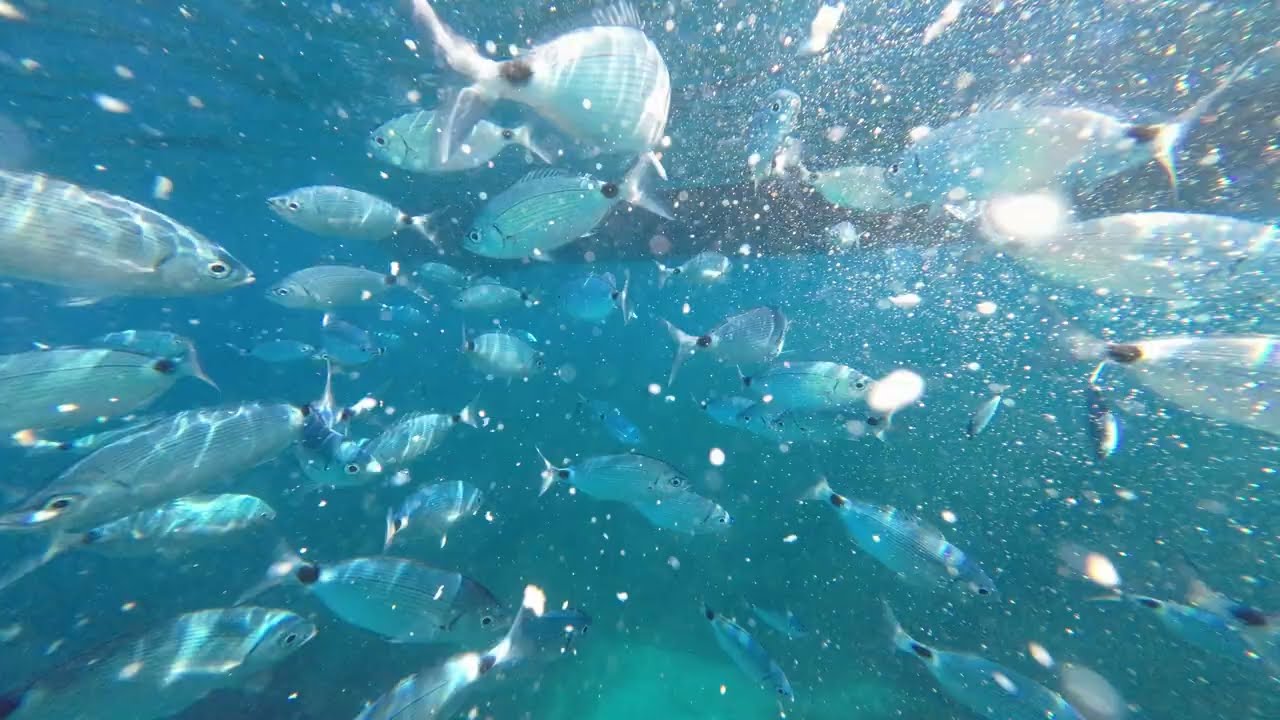This underwater photograph captures a large, vibrant school of fish swimming together in a turquoise sea, possibly the ocean. The fish are predominantly white to silver with flecks of blue and yellow on their undersides, each adorned with a distinctive black spot at the base of their tail fins. The water appears a bit murky with a greenish-blue hue, accented by tiny specks that could be plankton or debris, contributing to the dynamic movement visible in the scene. The image offers a view from behind the school, with the fish collectively swimming in one direction, creating a sense of unified motion despite their individual trajectories. The scene is set about six feet below the surface, where the sunlight filters through, illuminating the sandy, coral-strewn ocean floor. Amidst the fish, there is also a notably round, white fish adding to the diversity within the school. The presence of bubbles and movement within the water further enhances the sense of being surrounded by this lively aquatic environment.